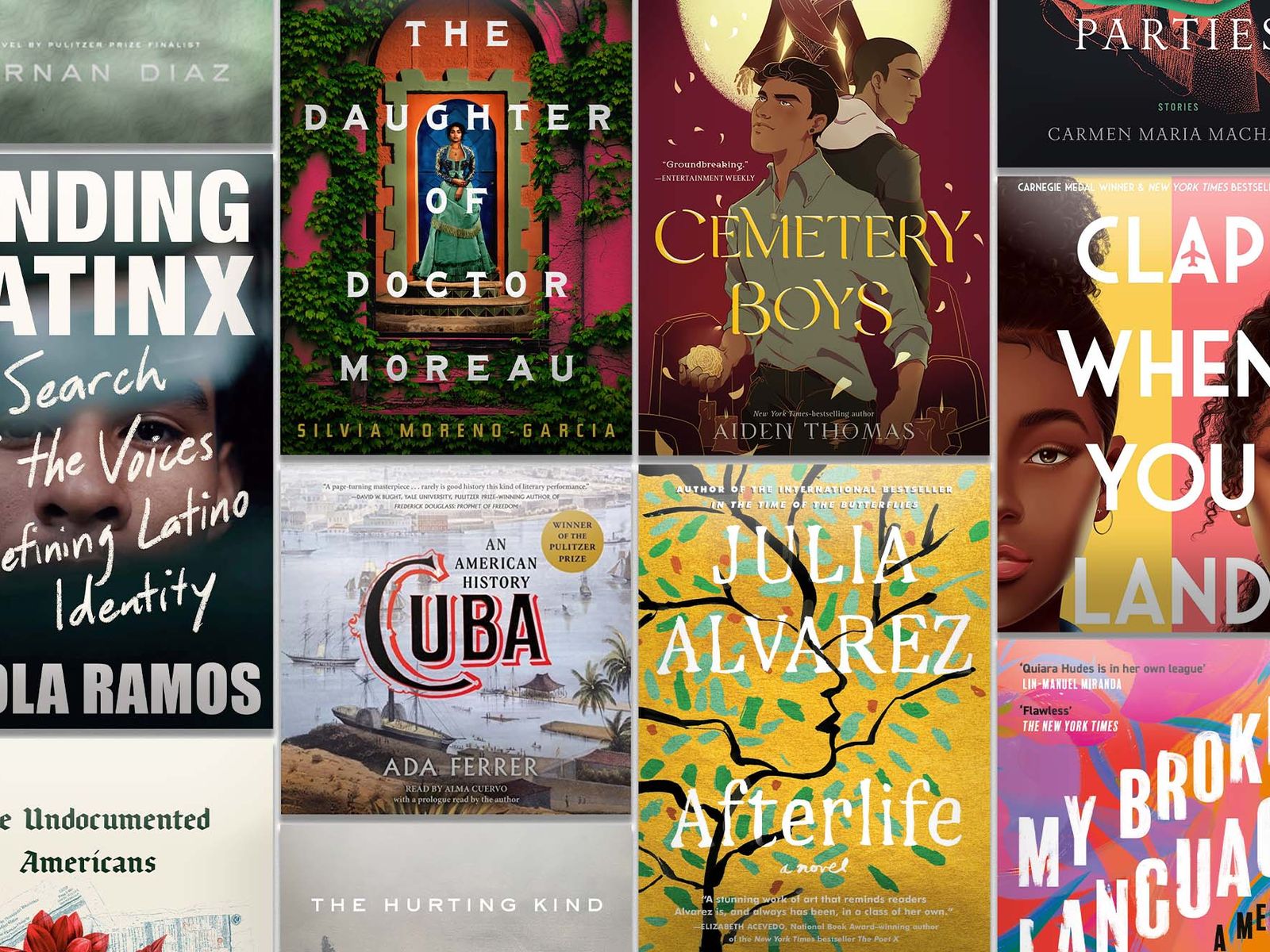This image is a detailed collage of various book covers, displayed in a vertical mosaic separated by thin, white lines. The arrangement is somewhat random, resembling a slot machine layout rather than a structured grid. The collage includes around nine books, many of which are by Latino authors or feature Latino themes. Notable titles include "The Daughter of Dr. Moreau" by Silvia Moreno-Garcia, which showcases a distinctly animated cover; "Cemetery Boys" by Aiden Thomas, another animated cover; "Clap When You Land," featuring two girls on the cover; "Afterlife" by Julia Alvarez, with a yellow background and illustrated tree branches; and "American History: Cuba" by Ada Ferrer, depicting an ocean scene with boats and palm trees. The diversity in cover designs includes a vibrant mix of colors such as pinks, reds, yellows, greens, whites, and grays. Some book titles are partially obscured, but notable mentions also include "Finding Latinx: In Search of the Voices Redefining Latino Identity" and "The Undocumented Americans," rounding out the eclectic array of books in this visually engaging collage.